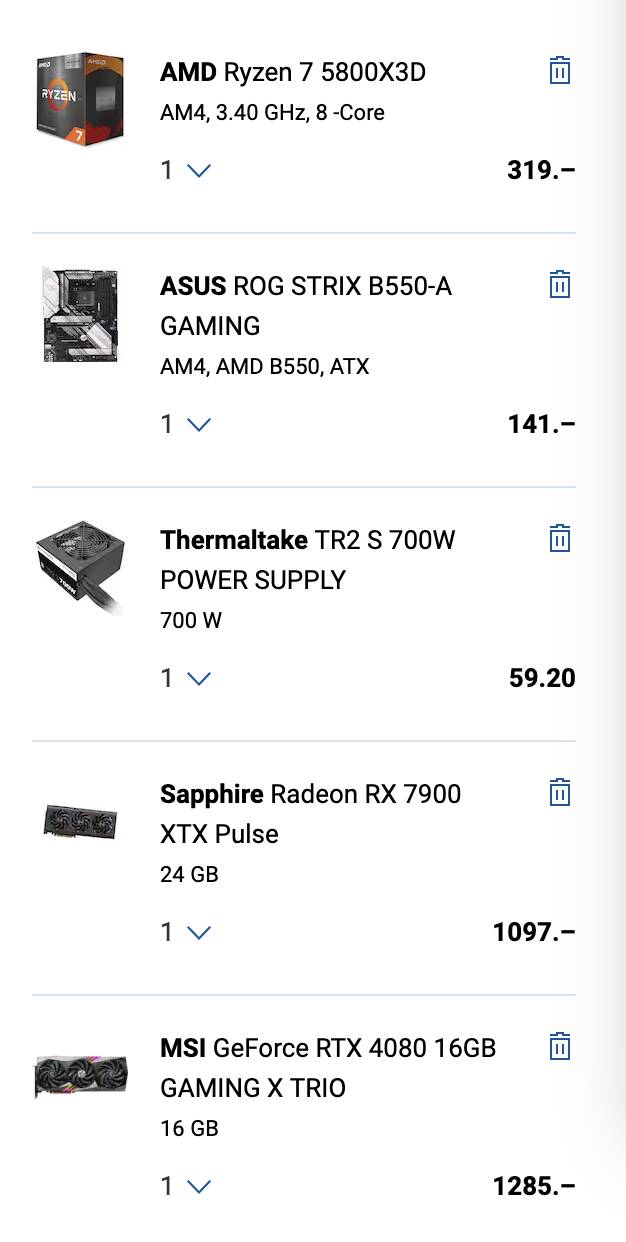In the image, there is a vertical arrangement of five products. Each product is listed with its corresponding name and company in a structured layout. On the left side, running from top to bottom, are images of the products. Adjacent to each image on the right side are the names and companies listed sequentially. The top product is from AMD, named Ryzen 7 5800X 3D. Below it is ASUS with the ROG STRIX-B550-A Gaming motherboard. Following that is Thermaltake’s TR2-S700W Power Supply, then Sapphire’s Radeon RX 7900 XTX Pulse graphics card, and finally MSI’s GeForce RTX 3080 16GB Gaming X Trio graphics card.

Continuing to the right of the product names are a series of numbers. For the AMD Ryzen 7 5800X 3D, the number 319 is listed. Below that, corresponding to the ASUS motherboard, is the number 141. Next to the Thermaltake power supply is the number 5920. The Sapphire graphics card is paired with the number 1097, and the MSI graphics card shows the number 1285.

Above these numbers on the far right, there is a light blue trash icon. The entire background of the image is white, with a light gray strip along the very right edge.